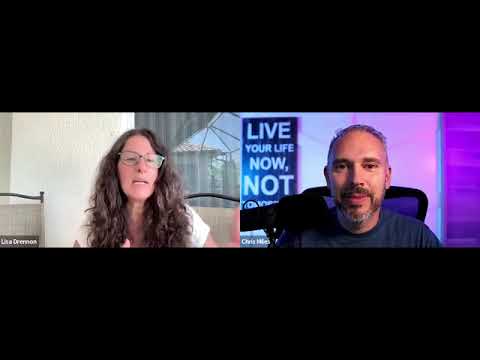The square image features a central horizontal strip displaying two individuals in separate sections, each framed by thick black borders at the top and bottom. The scene resembles a split-screen format frequently seen in video calls, suggesting the pair might be conversing through a platform like Zoom. On the left side is a woman with glasses and long, curly blonde-brown hair, wearing a white short-sleeve shirt. She appears to be speaking, with her mouth slightly open, and her portion of the image cuts off at her chest, revealing a white wall and a glass door behind her, possibly indicating she is sitting indoors near a window with curtains. 

On the right is a man with short, salt-and-pepper hair, a brown mustache, and a mostly gray beard. He is dressed in a dark t-shirt, also cropped at the chest. His background includes a light-colored wall, some neon lighting, and a significant black microphone obstructing part of a blue sign that reads in all caps, "LIVE YOUR LIFE NOW, NOT" with the rest cut off. The man’s setting suggests he might be in a studio, perhaps indicating he is hosting a podcast or participating in a professional recording. Both individuals are facing forward, creating the impression of direct engagement with the viewer. The detailed visual cues and the split-screen format evoke an organized, professional interaction.